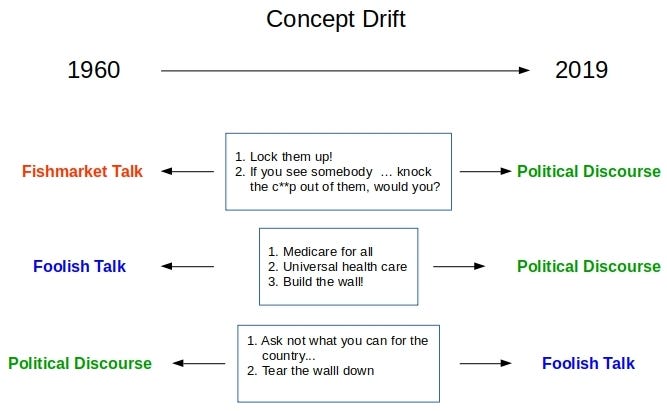The image displays a horizontal diagram titled "Concept Drift" at the top in black font. Below this title, an arrow stretches from "1960" on the left to "2019" on the right. The diagram illustrates how certain phrases have shifted in their perceived context over time through three horizontal rectangles.

The first rectangle lists:
1. "Lock them up!"
2. "If you see somebody...knock the C**P out of them, would you?"

To the left of this rectangle, an arrow labeled "Fish Market Talk" in orange-brown font relays the context for 1960, while an arrow on the right, labeled "Political Discourse" in green font, shows the context for 2019.

The second rectangle contains:
1. "Medicare for all."
2. "Universal health care."
3. "Build the wall!"

An arrow on the left designates it as "Foolish Talk" in blue font for 1960, whereas the right-side arrow labels it as "Political Discourse" in green for 2019.

In the third rectangle, the text reads:
1. "Ask not what you can do for the country."
2. "Tear down the wall."

Here, the left arrow marks it as "Political Discourse" in green for 1960, while the right arrow indicates it as "Foolish Talk" in blue for 2019.

The diagram visualizes the evolution of rhetoric over time, demonstrating how certain statements from 1960, initially marked as "Fish Market Talk" or "Foolish Talk," have transformed into "Political Discourse" by 2019, and vice versa.